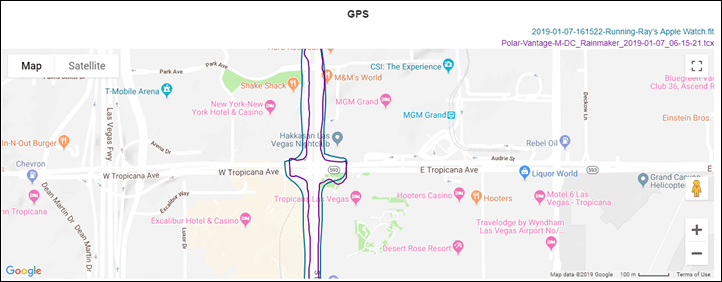The image is a screenshot of a GPS map centered around Las Vegas Fairway. The map displays an intricate network of roads, notably highlighting West Tropicana Avenue. Key landmarks and establishments are marked, including the Excalibur Hotel and Casino, Hooters Casino, Desert Rose Resort, Tropicana Las Vegas, MGM Grand, M&M World, Shake Shack, and an In-N-Out Burger.

Overlaying the map, there are hand-drawn annotations featuring a teal and a purple line. The teal line, labeled "2019-01-07 Running Ray's Apple Watch Fit," encircles an area at an intersection, while the purple line, labeled "Polar Vantage, Rainmaker," is placed within the teal boundary, both seemingly hand-drawn rather than digitally rendered. The map interface also shows control icons on the lower right corner, including a plus and minus sign for zooming in and out, respectively.